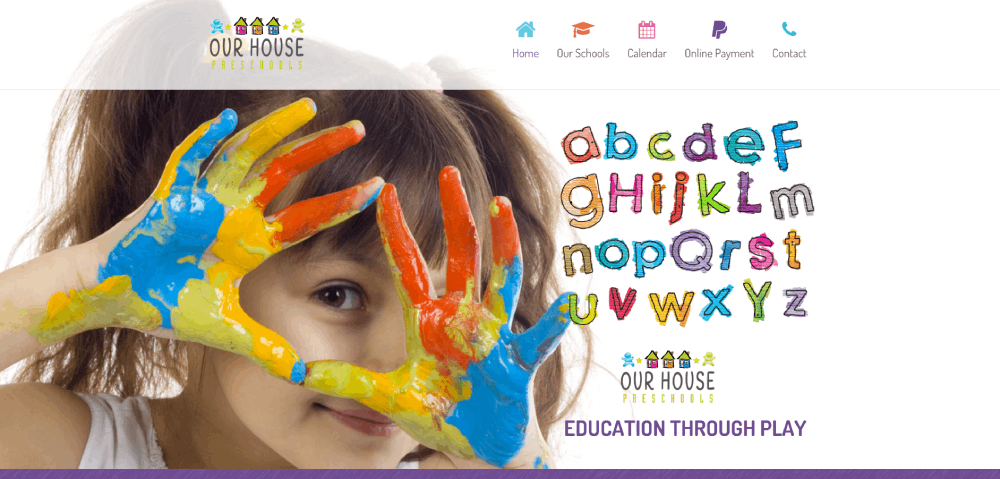The image depicts a detailed webpage layout for a preschool website called "Our House". Along the right-hand side of the page, there are several icons and labels including a house symbol for "Home," a hat icon labeled "Our Schools," a "Calendar" section, and an "Online Payment" area featuring the PayPal logo. Beneath these, there is a telephone icon accompanied by the word "Contact."

At the bottom of the page, there is a vibrant image of a young girl, presumably a preschooler, with light skin, brown hair styled in pigtails with bangs, and brown eyes. The girl has her hands raised and is peering through them, displaying brightly colored paint, suggesting she has been finger painting. 

Adjacent to this image, the alphabet (A to Z) is displayed in a playful, crayon-colored style. Below this, the text "Our House Preschool" is prominently featured, along with a house icon and a group of children, underscoring the theme of community and education. Following this is the phrase "Education through Play," emphasizing the preschool's educational philosophy.

At the very bottom of the screen, there is a long, thin purple bar, which likely serves as a website footer. Overall, the webpage is visually engaging and indicative of a preschool environment focused on playful learning and community.